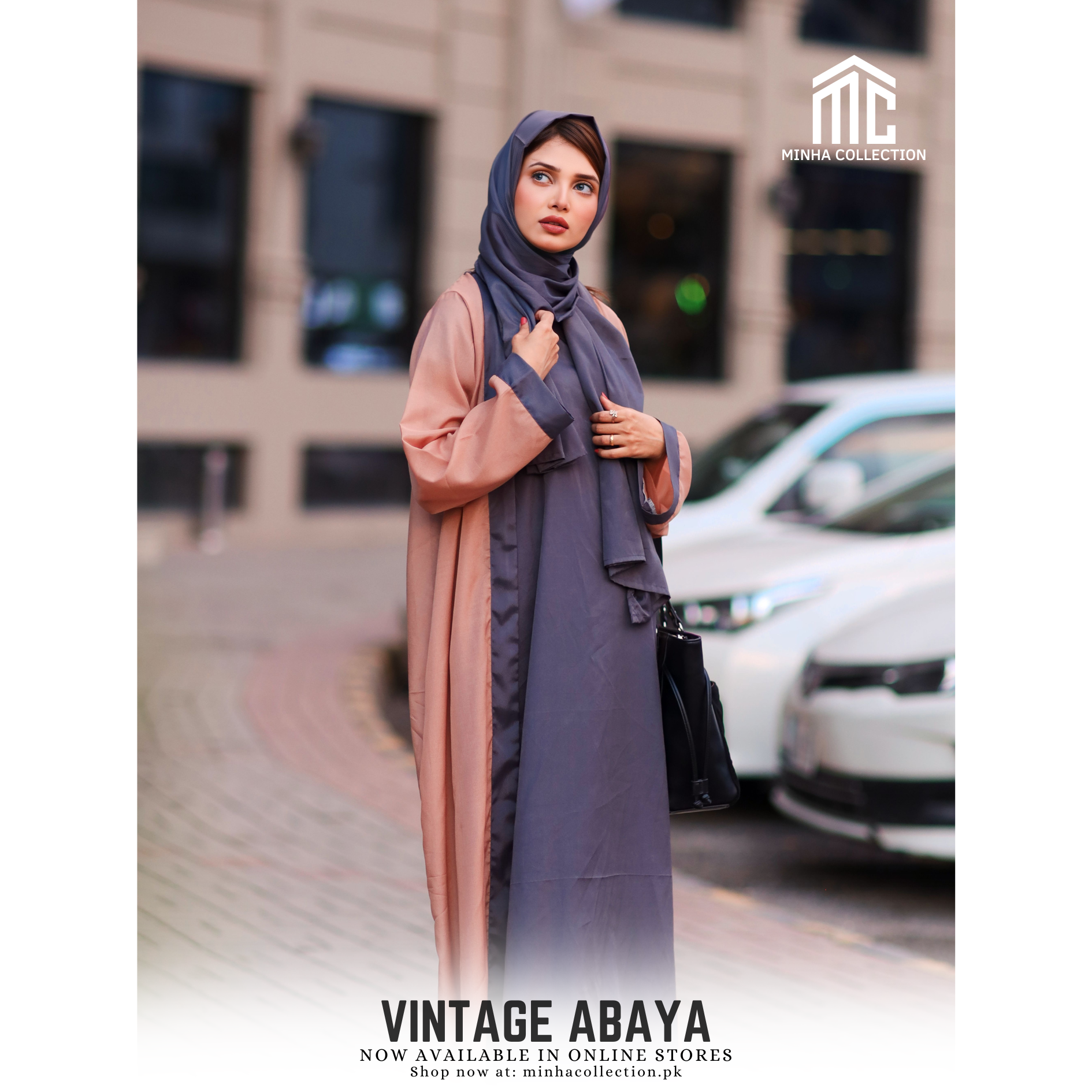This detailed fashion photograph, possibly enhanced with a filter, features a model showcasing a Vintage Abaya from the Minha Collection. The top right corner of the image displays a white logo with the letters "MC" and a triangular roof above them, along with the brand name "Minha Collection." The bottom of the image reads, "Vintage Abaya, now available in online stores. Shop now at minhacollection.pk."

The background is blurred, consisting of light tan buildings and three white cars, placing the focus on the model. She stands in front of a building, with a stone positioned directly below her. The woman is light-skinned with brown hair peeking out from under a bluish-purple, wraparound scarf that drapes elegantly down to her feet. She is adorned in a matching mauve-pink robe, detailed with dark gray cuffs. 

Her makeup is meticulously done, featuring striking red lipstick. She carries a black leather bag to her side and showcases her manicured red nails. On her left hand, she wears multiple rings. She gazes upwards, adding an air of sophistication and poise to the overall composition.